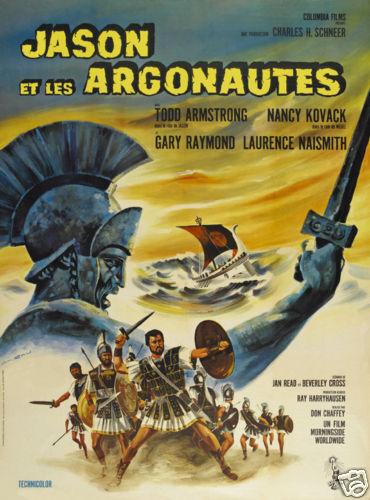This image is an intricately detailed movie poster for "Jason et les Argonautes," the French version of the classic film. The title, displayed prominently in bold yellow at the top, reads "Jason A. Les Argonauts." Dominating the visual space, a massive stone statue of a warrior wearing a Roman helmet holds a sword aloft, commanding attention. At the center of the poster, a boat battles through rough, tumultuous waves, emphasizing the epic scale of the adventure. In the foreground, a contingent of Roman troops, donned in traditional armor and crested feather helmets, stand ready for battle. One soldier, clad in an armored vest and Roman tunic, stands at the forefront with a circular shield, leading the charge. The poster also lists the prominent actors in the film: Todd Armstrong, Nancy Koyak, Gary Raymond, and Lawrence Naismith, hinting at a star-studded cast bringing this legendary tale to life.